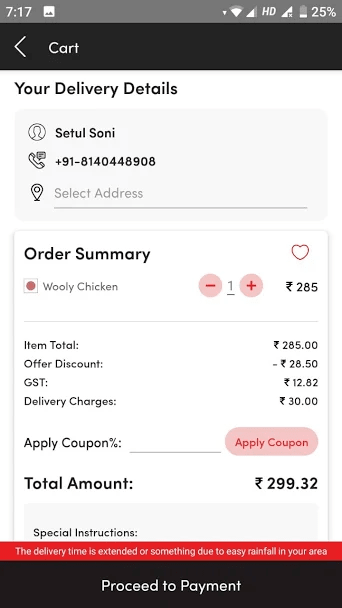At the top of the image, there is a very thin gray strip. On the left side of this strip, it displays the number "717". Towards the right, there is a white image icon. Further to the right, you can see a Wi-Fi symbol and a cellular data signal indicator, marked with the letters "HD" in an italicized font. To the right of these indicators, there is another data signal icon with an "X" at its bottom right corner. Following this is a battery icon, approximately one-quarter filled, with the inscription "25%" in white.

The next section features a header that is about three times larger than the thin gray strip above. This header has a black background. On its left side, there is a white arrow pointing to the left, adjacent to the word "CART," which is written in a font reminiscent of Century Gothic in white lettering.

Beneath this header, the background transitions to white. In bold black font, the text "Your Delivery Details" is displayed. Below this, there is a rectangular area with rounded edges, filled with a light gray background. Inside this area, a user icon is present within a circle outlined in black. Adjacent to the icon, the name "S-E-T-U-L-S-O-N-I" is written in bold lettering. Additionally, a phone icon is shown within a message bubble extending from the center of the phone icon, indicating the phone number "+91-814-044-8908."

Underneath the user details, on the left side, there is a black map pin icon. To the right, there is a field enabling address selection, labeled "Select Address" in light gray text. Below this, there is a rectangular shape with a shadowed gray border. In the top left corner of this rectangle, the words "Order Summary" appear in bold black lettering.